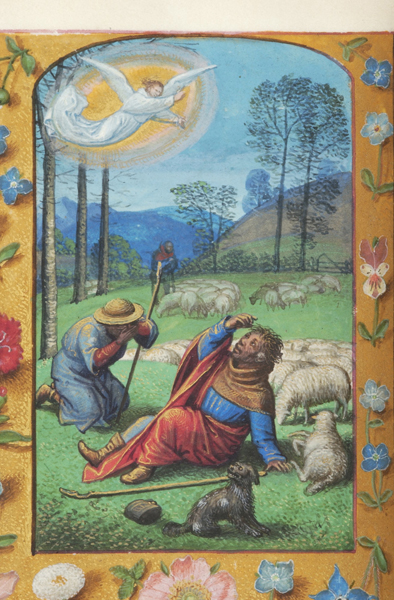This vivid illustration, seemingly inspired by biblical themes and executed in an older artistic style, vividly captures a serene pastoral scene. Central to the composition is a mystic encounter between humble shepherds and a celestial being. A radiant angel with white wings and a flowing white robe, adorned with red hair pulled back in a bun, floats overhead in a brilliant halo of yellow light above a bright blue sky. 

Below, in lush green grass, a shepherd in a blue robe with a red wrap and brown shawl, sits on the ground shielding his eyes in awe, his shepherd’s crook lying nearby. Another shepherd in a similar blue robe and straw-colored hat kneels with his hands over his face, overcome by the divine sight. A standing shepherd can be seen in the background, adding to the sense of reverent wonderment.

The scene is populated by a collection of plump, woolly sheep, approximately thirty in number, all gazing towards the miraculous vision. Among them, a single black dog also directs its attentive gaze upwards. The pastoral setting is framed by a landscape of rolling blue hills and distant mountains, adding depth and serenity to the scene. Encircling the entire tableau is a decorative border adorned with yellow and small floral motifs, enhancing the illustration with a touch of quaint charm.